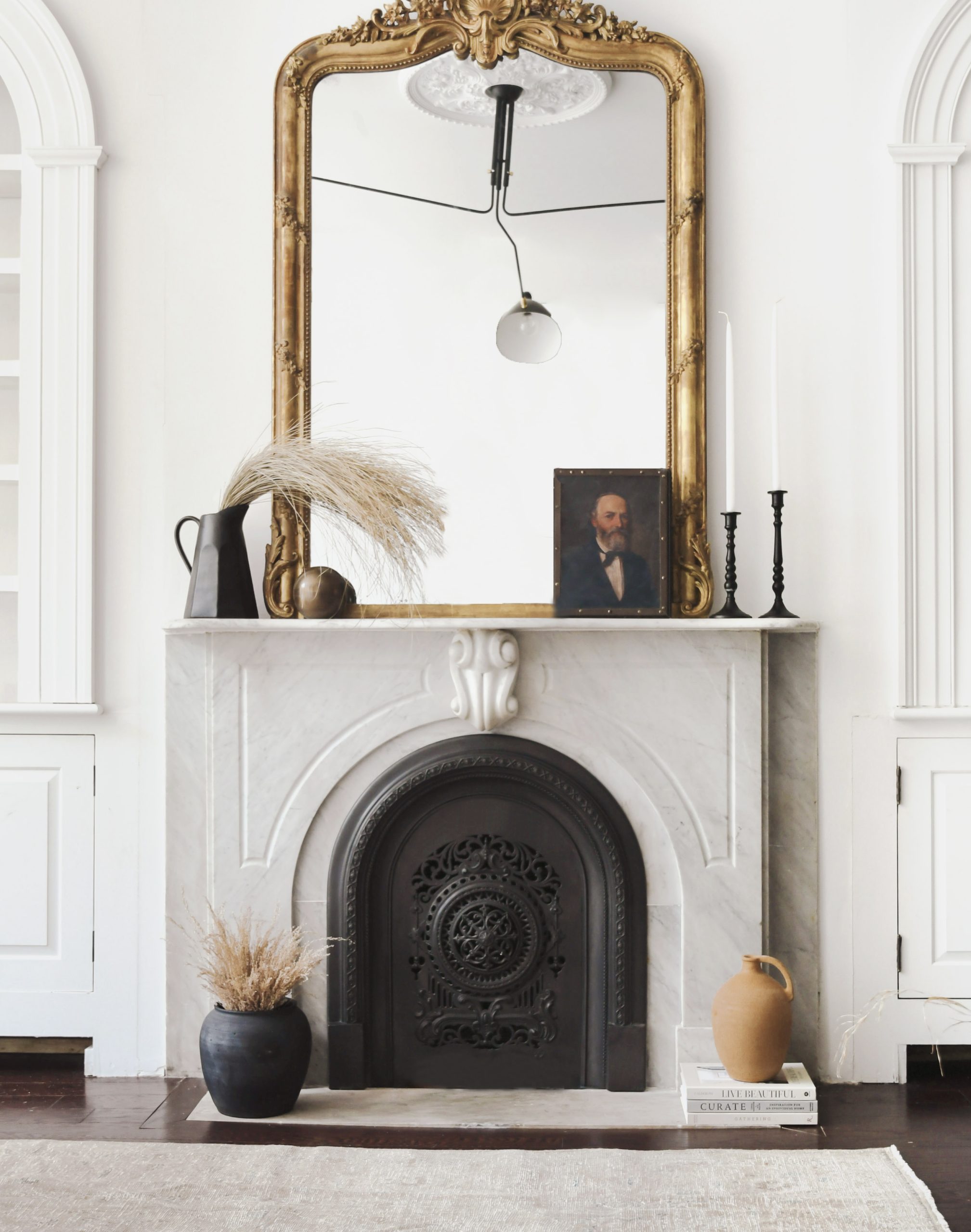This image captures a cozy, indoor setting featuring a detailed view of a fireplace, likely in a living room. The fireplace is framed by a white marble arch and has a decorative black metal grate adorned with an ornate circular design at its center. Positioned on the fireplace mantle, from left to right, are a black pitcher with dried flowers resembling wild grass or wheat, an old-style photograph of a man in a suit with facial hair, and black candlesticks with white candles. Dominating the center of the mantle stands a large, ornate mirror with a brass border, reflecting a hanging lamp from the ceiling. Flanking the base of the fireplace are two pots: on the left, a black pot containing brown, dry plants, and on the right, a tan jug styled as an old-time vase. The scene is set against a white-walled background, and the colors present include white, black, tan, beige, brown, and gold. The room features wood flooring and a carpet, adding to the warm, inviting atmosphere.